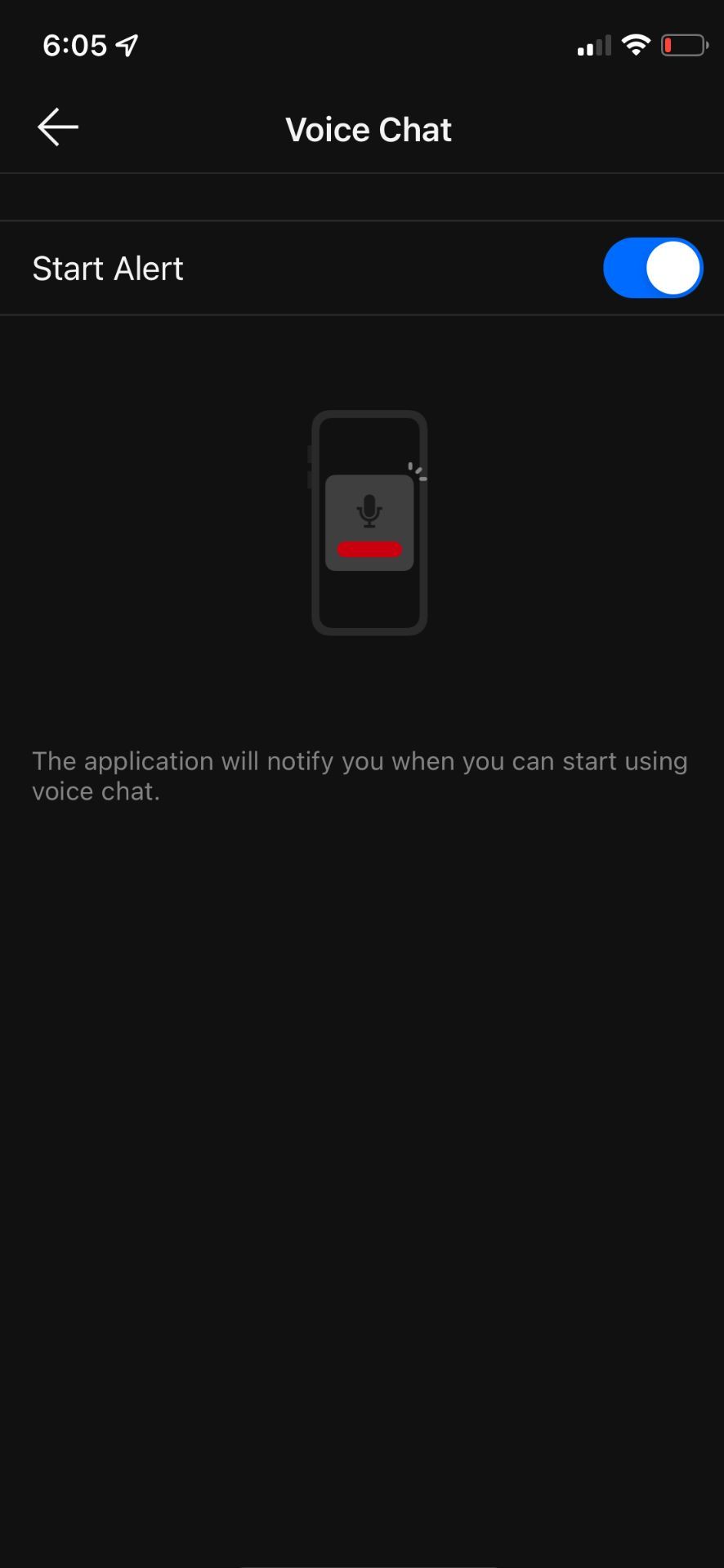The image displays a graphical interface of an iPhone set to dark mode, illustrating the "Voice Chat" feature. At the top of the screen, the phrase "Voice Chat" is clearly visible. Directly below this, towards the left, there is an option labeled "Start Alert" accompanied by a slider button on the right, currently toggled to the right.

Beneath this setting, a small silhouette of a cell phone is shown, featuring a horizontal red bar below the microphone icon. This indicates the notification status of the application. Further down, there is a message stating, "The application will notify you when you can start using voice chat."

The purpose of this graphic is to highlight the location and functionality of the "Start Alert" slider button for the voice chat feature. The iPhone is in dark mode, resulting in a predominantly black background. Additionally, the status bar at the top reflects the time as 6:05 and indicates a low battery. The lower half of the image is entirely black, devoid of any icons, messages, text, or other overlays. The graphic serves solely to demonstrate the activation of the "Start Alert" option within the voice chat settings.